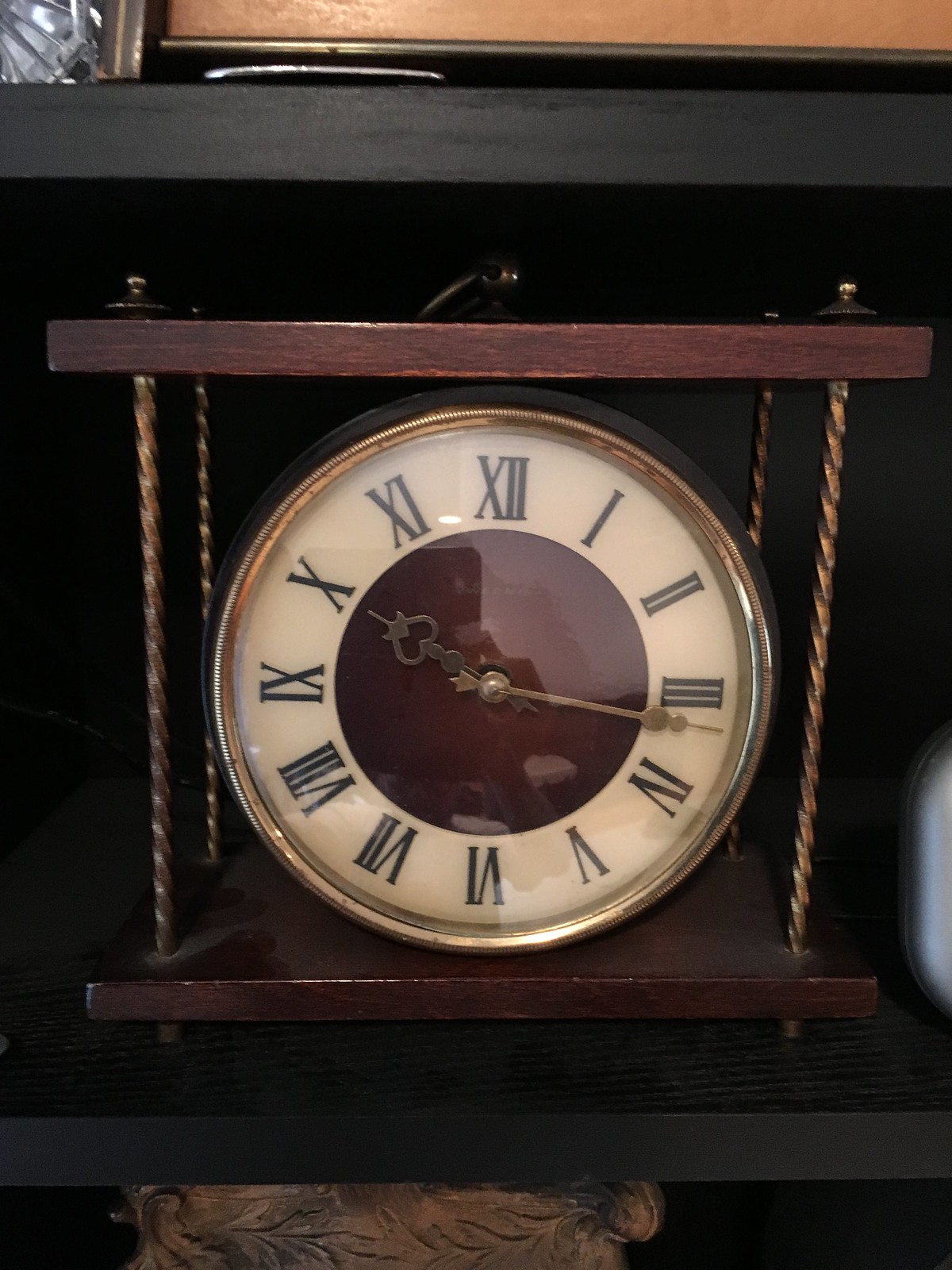This image showcases an elegant mantel clock encased in a distinguished design. At the top, there is a piece of rich burgundy-brown wood, accompanied by four goldish-bronze rods that extend downward to a matching wooden base. The wooden components are joined with visible bolts, contributing to its vintage aesthetic. The top of the structure features a small handle made from the same metallic material as the rods.

The clock itself is encircled by a black border that frames a gold ring around the clock face. The off-white face of the clock displays classic black Roman numerals from I to XII. At the center, a prominent burgundy circle houses the delicate gold hour and minute hands. The clock face is protected by a glass cover, which may either be bubbled or flat—it's difficult to ascertain.

This refined timepiece sits on a black shelf, part of a larger furniture piece that also has additional brown components around it. This shelf and the potential cabinet or surface beneath it seem to be made of wood, contributing to the overall sophisticated and antique appearance of the setting.